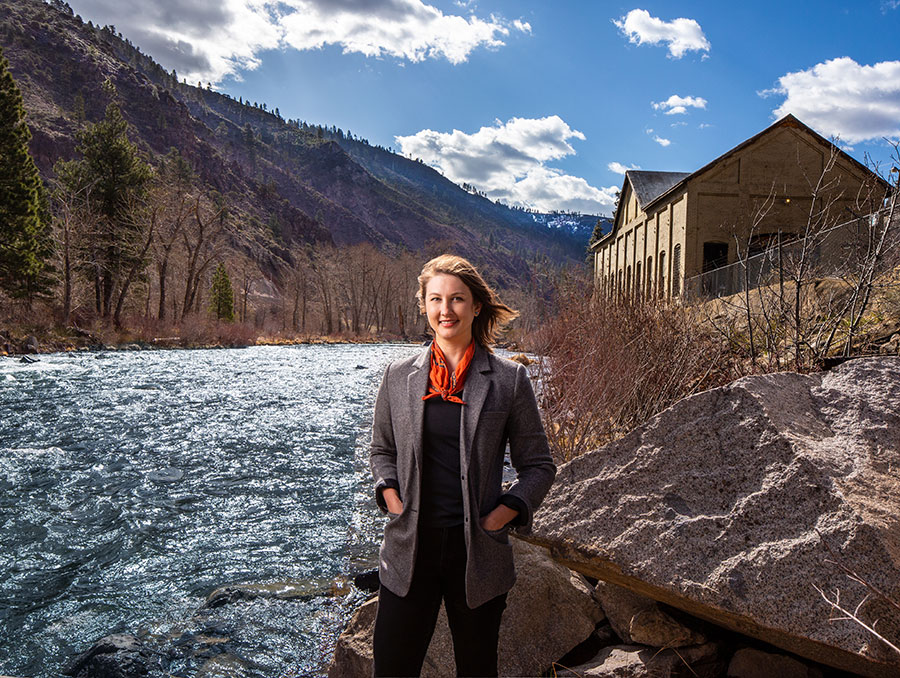In this detailed image set outside during the day, a woman stands confidently on jagged rocks by a fast-flowing river, her pose suggesting it could grace the cover of a magazine. With short blonde hair tousled by the wind, she wears a gray blazer over a black shirt and black pants, accented by a vibrant red scarf tied around her neck. Her hands rest in her pockets as she smiles, her gaze directed forward. To her left, the river courses swiftly, flanked by a mountain covered in bare and some green-leafed trees. On the right side of the image, the hillside she stands by is dotted with brown, leafless bushes. A large, brown building with numerous windows looms in the background atop the hill. The scenery is under a mix of cloudy and blue skies, completing the picturesque setting that, despite its realistic appearance, hints at digital enhancement.